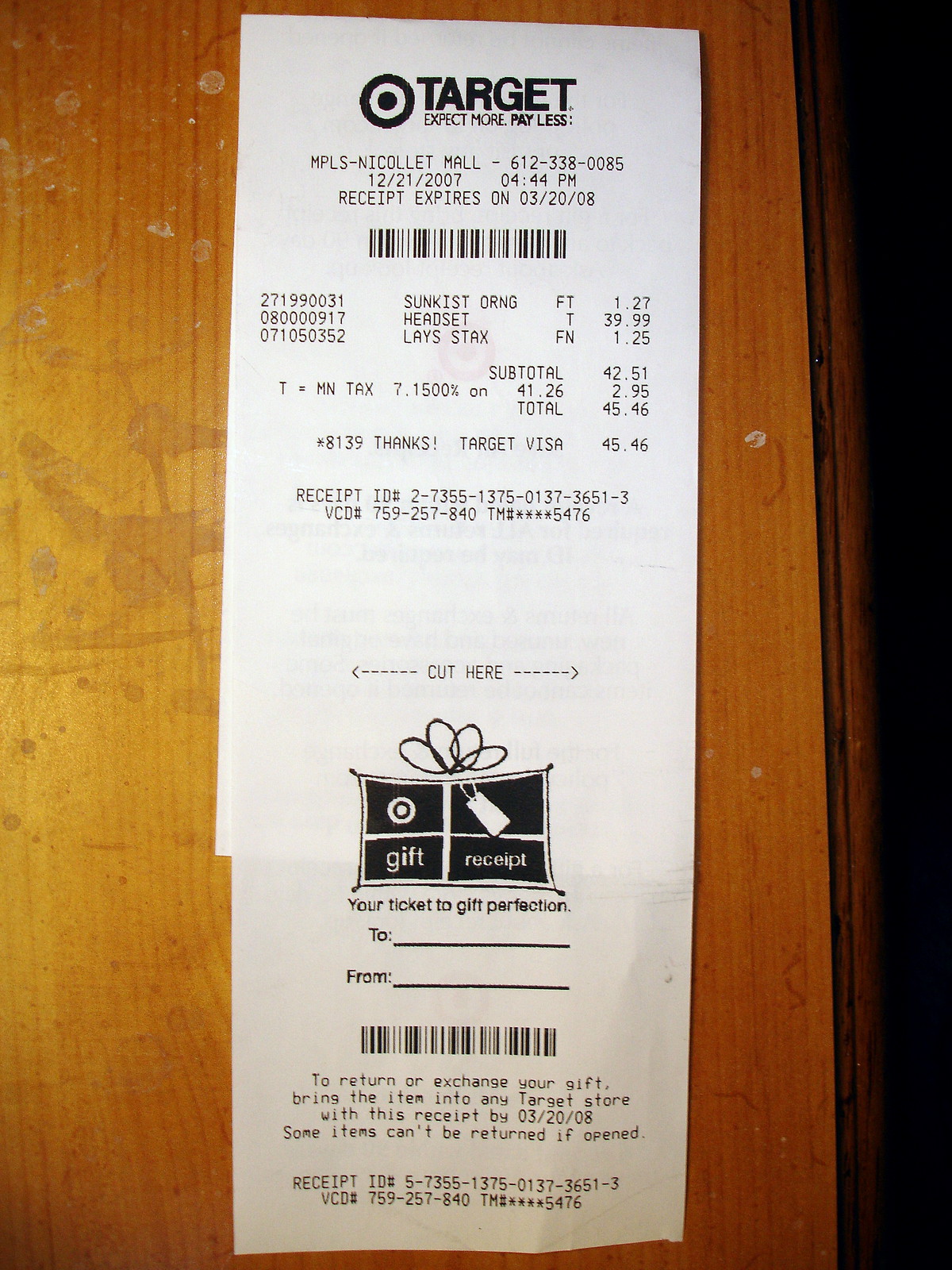This image features a detailed receipt placed on top of a wooden desk. The receipt is from a Target store located at Nicollet Mall, with a store number of 612-338-0085. It indicates that the payment was made using a Visa card ending in 8139, and highlights that the transaction took place in Minnesota, as shown by the "MN Tax" notation. The state tax rate applied is 7.15%.

The total amount spent was $45.46, which included the purchase of a sun-kissed orange, a headset, and Lays Stacks. The transaction date and time are provided as December 21, 2007, at 4:44 PM. Additionally, the receipt mentions an expiration date for returns or exchanges, set for March 20, 2008. Instructions for returns are clearly stated, advising customers to bring the item to a Target store along with the receipt within the specified period. The receipt's format appears standard, containing all typical retail transaction details.